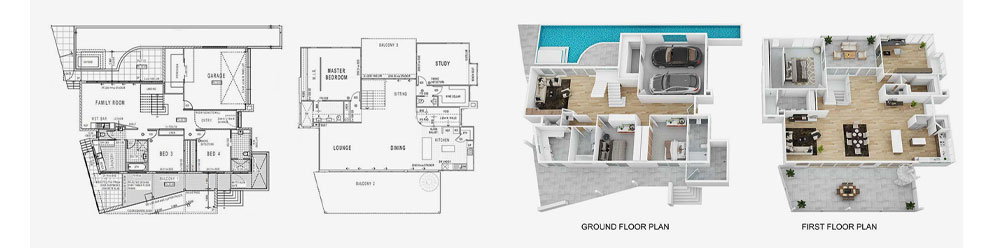The rectangular image portrays a detailed layout of a building in four distinct sections, with a light gray background. It spans about five inches wide and an inch high. On the far left, there is a small black and white pencil drawing illustrating what appears to be the ground floor, including rooms such as the garage, family room, and bedrooms three and four. Text on this drawing is difficult to decipher due to its small size. 

Next to the leftmost image is another black and white illustration, slightly clearer, depicting the second level of the building. Here, labels like master bedroom, bedroom one, study, lounge, and dining area can be identified. 

To the right of the black and white sketches, there is a colored image indicating the ground floor plan. This section features detailed additions like a black car and a silver car in the garage, a pool adjacent to the house, and labeled wooden floors. 

The final section on the far right is also in color and depicts the first floor plan, complete with detailed furniture arrangements. Notably, the balcony, located below the lounge, is furnished with a central table surrounded by three plants in various corners and an additional table in the top right corner. This comprehensive layout gives a meticulous view of the building's design, combining basic blueprints and colored 3D renderings of both floors.